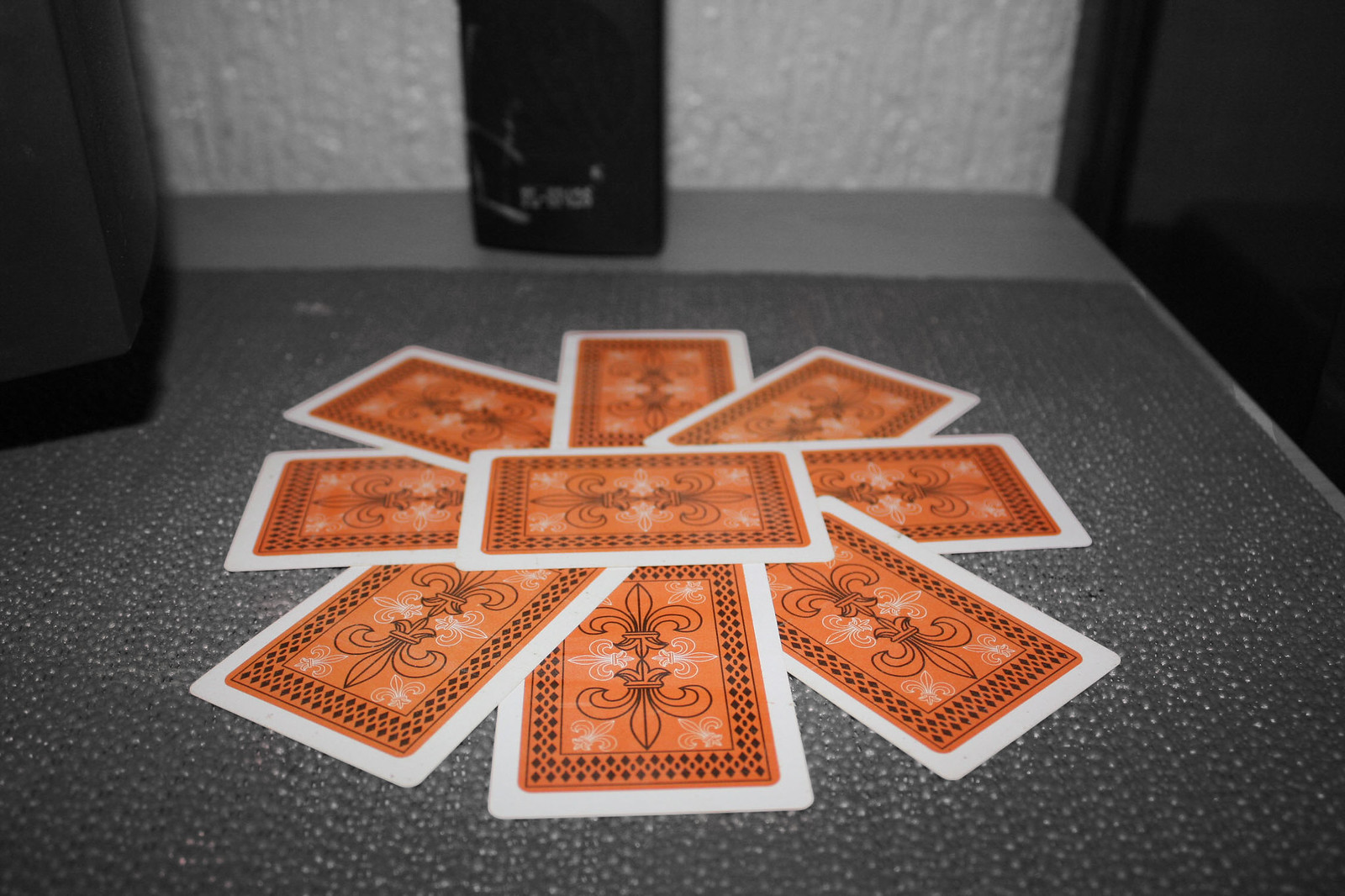The photo is captured in landscape mode on a textured gray tablecloth that rests atop a gray counter. The center of the composition is dominated by nine playing cards, arranged in a star-like asterisk pattern. Each card features a white border, an orange background, and an internal diamond-shaped border. Within each diamond, two black fleur-de-lis symbols are centrally placed, accompanied by four smaller white fleur-de-lis symbols pointing inward from the corners. The background of the photo includes three indistinct plastic objects, too blurred to identify. The backdrop comprises a heavily textured white wall, with the table positioned adjacent to a sleek, shiny black surface—potentially a door or appliance, though the close-up nature of the image leaves this detail ambiguous.